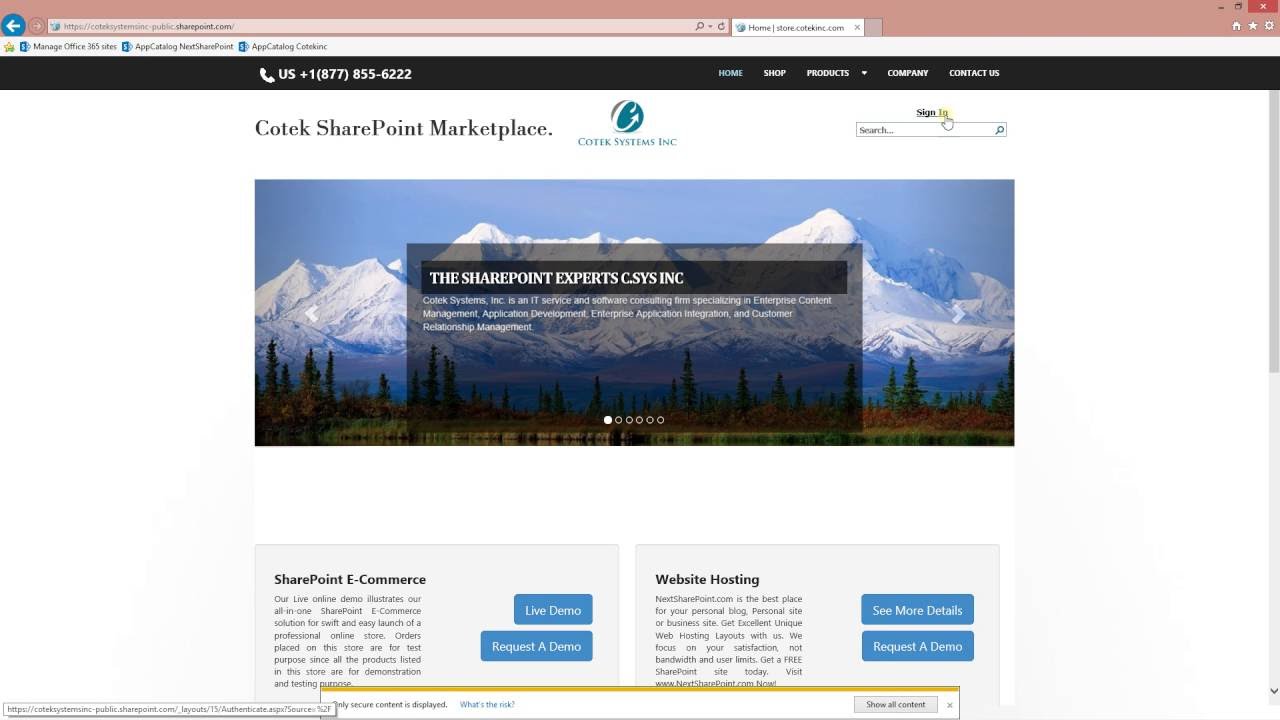**Detailed Caption:**

This is a detailed screenshot of the *Cortex SharePoint Marketplace* website. The top of the webpage features a prominent orangey-pink bar with a distinct blue-black button. Beneath this bar is a black strip housing a search box and a phone number, with some tiny text aligned to the right side. The background of the page is predominantly white with black text, providing a clean and professional look.

Centrally placed on the page is the *Cortex SharePoint Marketplace* logo, characterized by its white and blue colors. A search box is located on the right, adjacent to a sign-in box icon featuring a small hand cursor.

Dominating the center of the screenshot is a scenic image of mountains with trees in the foreground and a clear blue sky. Superimposed on this image is a semi-translucent grey box with white text, which reads, “*SharePoint Experts CSSIS Inc.*” This description details that *Codex Systems Inc.* is an IT service and software consulting firm with expertise in enterprise content management, application development, enterprise application integration, and customer relationship management.

Below this text, there is a row of six circles; the first circle is solid white, while the remaining five are outlined in white.

Lower on the webpage, the screenshot highlights two main sections: *SharePoint e-commerce* on the left which offers options like "Live Demo" and "Request a Demo," and *Website Hosting* on the right, with similar options – "See More Details" and "Request a Demo." Beneath these sections are paragraphs that provide detailed information about each offering.

Finally, there is a pop-up bar at the bottom of the screenshot with a yellow edge at the top that warns, "Only secure content is displayed. What's the risk? Show all content." This pop-up ensures the user's awareness of the nature of the displayed content.

This image not only captures the layout and aesthetic of the website but also conveys the hierarchical structure and available functionalities in a clear and descriptive manner.